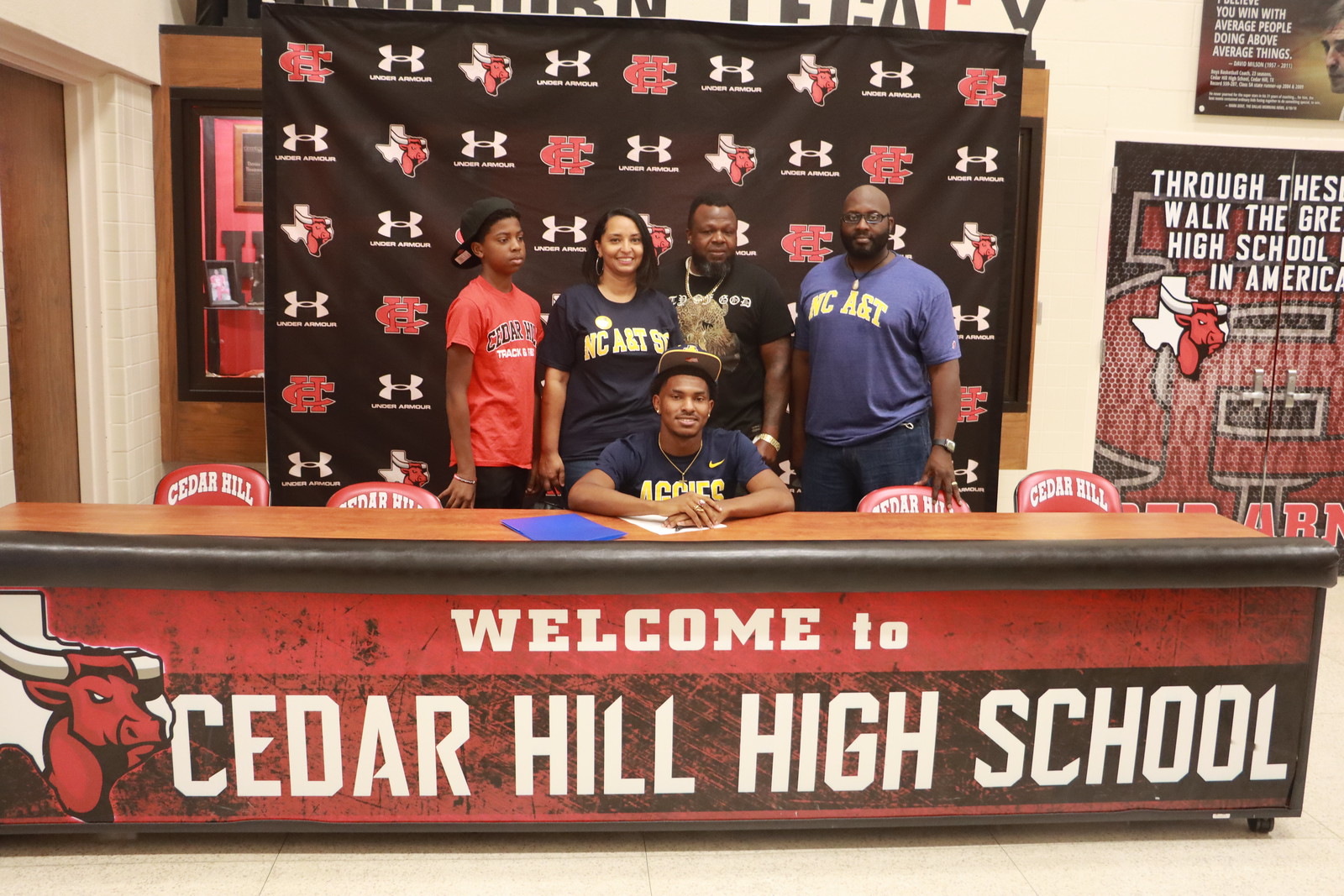In the image, there are five African American individuals, positioned indoors in what appears to be a high school setting, likely related to a school event or sports faculty meeting. Prominently featured in the foreground is a long, wooden counter displaying a red banner with bold text that reads, "Welcome to Cedar Hill High School," accompanied by the school mascot—a red bull with black horns.

Seated behind the counter is a young man wearing a black baseball cap, a black Nike t-shirt with yellow lettering, and a cross necklace. He is smiling and has a blue folder and a pen in front of him. Standing behind him, from left to right, are four people:

1. A young man wearing a backward black baseball cap, a red t-shirt with "Cedar Hill Track" lettering, and black pants.
2. A smiling woman with short hair, dressed in a black t-shirt with yellow lettering.
3. An older man with a black and gray beard, wearing a black t-shirt featuring gold chains and a gold necklace, with the word "God" visible on his shirt.
4. A bald man with a black beard, black glasses, a blue round-neck t-shirt with yellow lettering, dark blue pants, and a wristwatch.

The background includes a banner with multiple school logos, including a white "H" with "Under Armour," a red "HC" joined together, and a map background with an animal, possibly a bull. Visible in the background are doorways, a glass window, and motivational posters, one of which reads, "You win with average people doing above-average things," along with a partially visible banner continuing the school’s message.